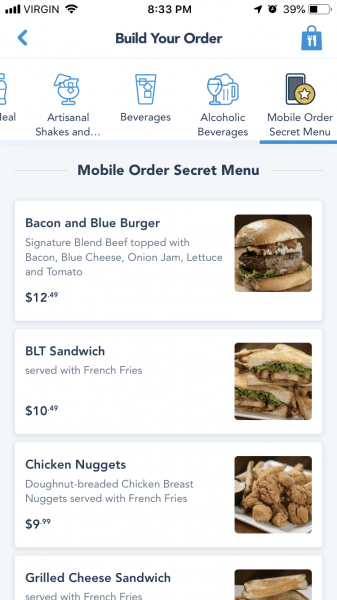Screenshot from a food ordering website: 

At the top of the screen, the status bar displays phone details, including a cellular network identifier "Virgin," a Wi-Fi symbol, the current time "8:33 p.m.," a location symbol, an alarm symbol, and a battery level at 39%. 

The main section of the screen is dedicated to the app, featuring a header that reads "Build Your Order." To its right is an icon of a cart representing the current order, while to the left is a back arrow for navigation. Below this header, a menu offers options segmented into categories: "Artisanal Shakes," "Beverages," "Alcoholic Beverages," and "Mobile Order Secret Menu," each accompanied by minimalist icons such as outlined glasses or beer cups.

The currently selected category is the "Mobile Order Secret Menu," listing multiple items:
1. **Bacon and Blue Burger:** A signature blend beef patty topped with bacon, blue cheese, onion jam, lettuce, and tomato for $12.49.
2. **BLT Sandwich:** Served with French fries for $10.49.
3. **Chicken Nuggets:** Donut-breaded chicken breast nuggets served with French fries for $9.99.
4. **Grilled Cheese Sandwich:** Served with French fries, though the price is partially cut off.

Alongside each menu item, there is a corresponding image providing a visual reference.